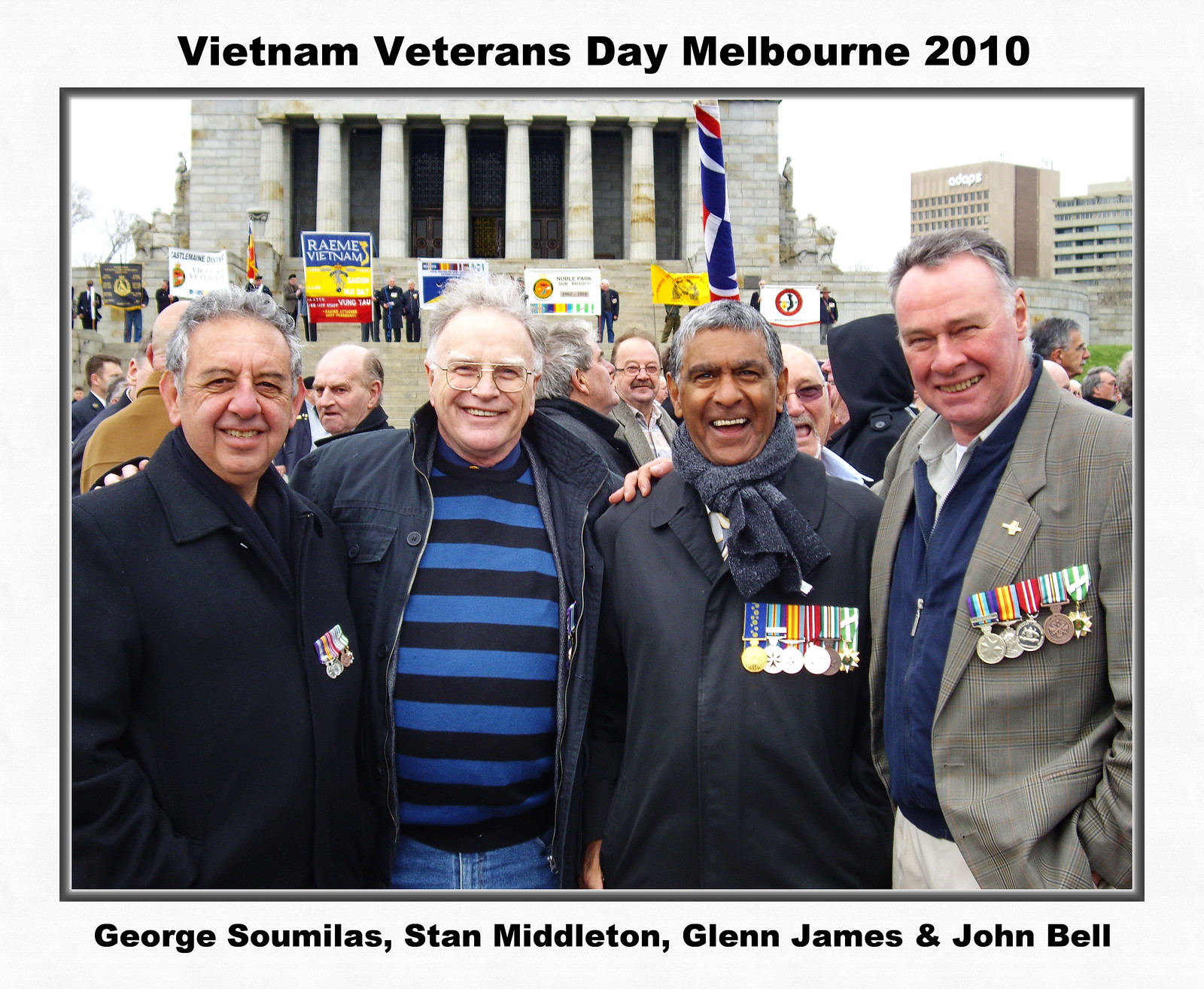The image features four men, identified as George Sumilis, Stan Middleton, Glenn James, and John Bell, standing close together in front of a grand stone building with large pillars, possibly a government or memorial structure. The caption above the photograph reads "Vietnam Veterans Day, Melbourne, 2010," indicating the event being celebrated. Beneath the photograph, their names are listed. The men appear to be in their 50s or 60s, with three of them sporting short gray hair and one having a darker complexion, possibly of Central Asian descent. They are dressed in regular attire adorned with military ribbons, smiling warmly at the camera with their arms around each other. The background is bustling with numerous people holding large signs and flags, adding to the festive, commemorative atmosphere of the event presumably related to the Vietnam War.